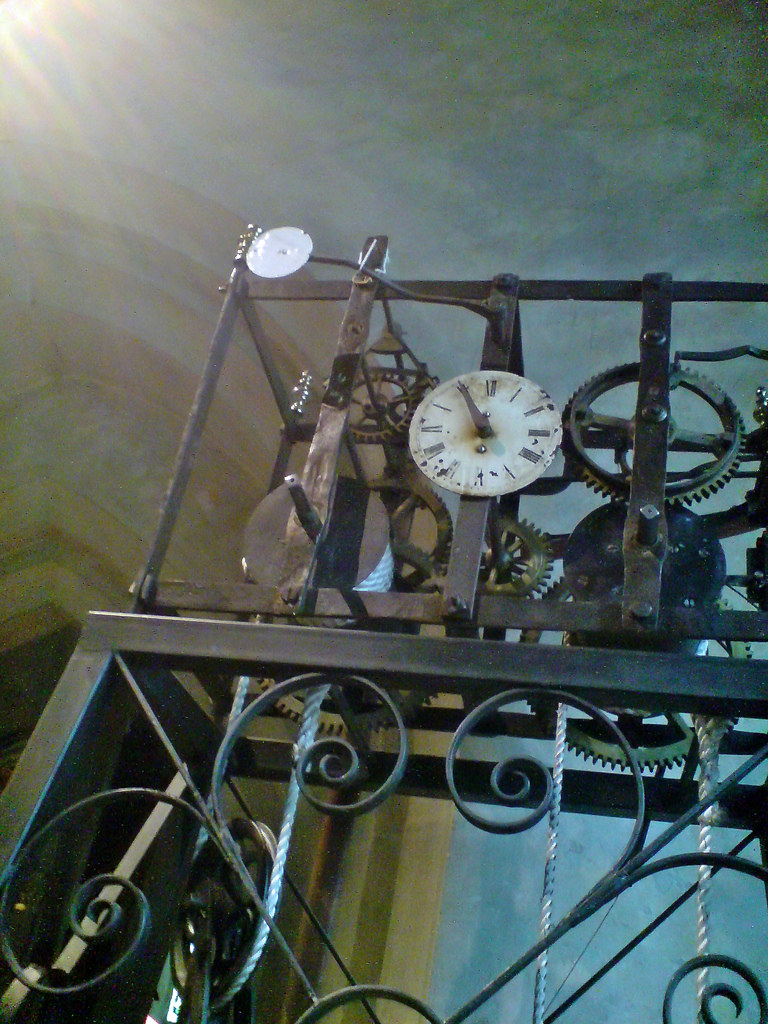The image depicts a detailed and intricate steampunk-looking mechanism viewed from below. The central feature is a clock encased in a rectangular metal frame with no sides, revealing a complex inner system of copper-colored gears and silver cables. The clock's face is white, albeit dirty and dusty, with black numbering and black hour and minute hands both pointing to 11. Beneath the clock, there is an elaborately designed wrought iron railing, resembling those found on porches, adorned with swirling patterns. Above it, the frame's top consists of a fence-like black metal structure. The background showcases a blue roof and wall, hinting at the setting's industrial aesthetic. The overall impression is of a deconstructed or partially assembled antique timepiece, rich in detail and history.